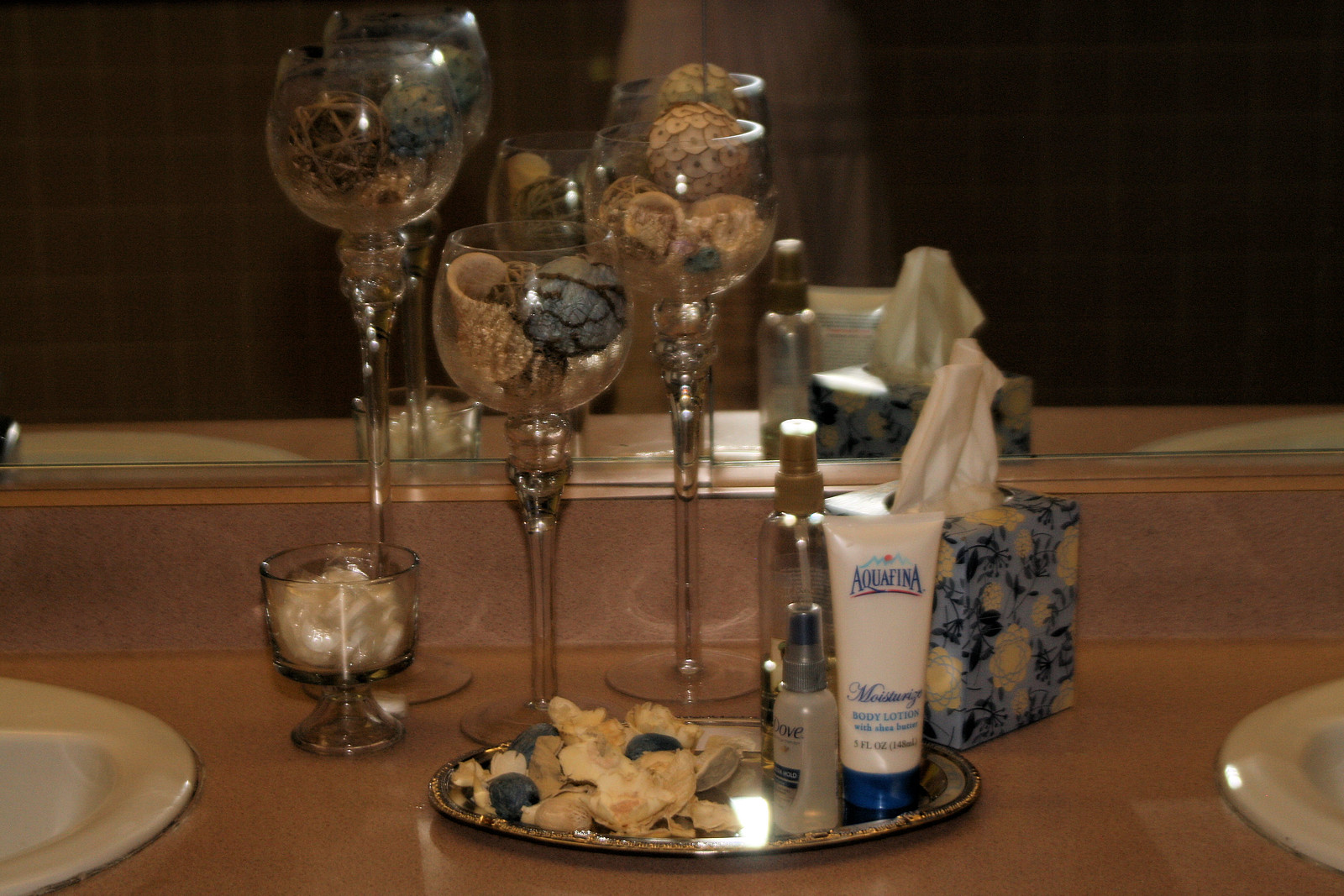A close-up image showcases a decorative bathroom sink setup. At the center of the brown countertop, there's a silver platter adorned with beige and blue trinkets. Adjacent to the platter are a few beauty products: a cream-colored bottle labeled "Aquafina Moisturizer Body Lotion," a small transparent spray bottle marked "Dove" containing a clear liquid, and another partially filled see-through bottle with a gold cap, though its label is unclear. Behind these items is a blue tissue box with a floral design and a tissue protruding from the top. Framing the scene are the edges of two sinks. Three tall-stemmed wine glasses, each filled with decorative items, and a smaller bell-shaped glass with a white object inside add an elegant touch. Reflecting the arrangement is a bathroom mirror in the background.